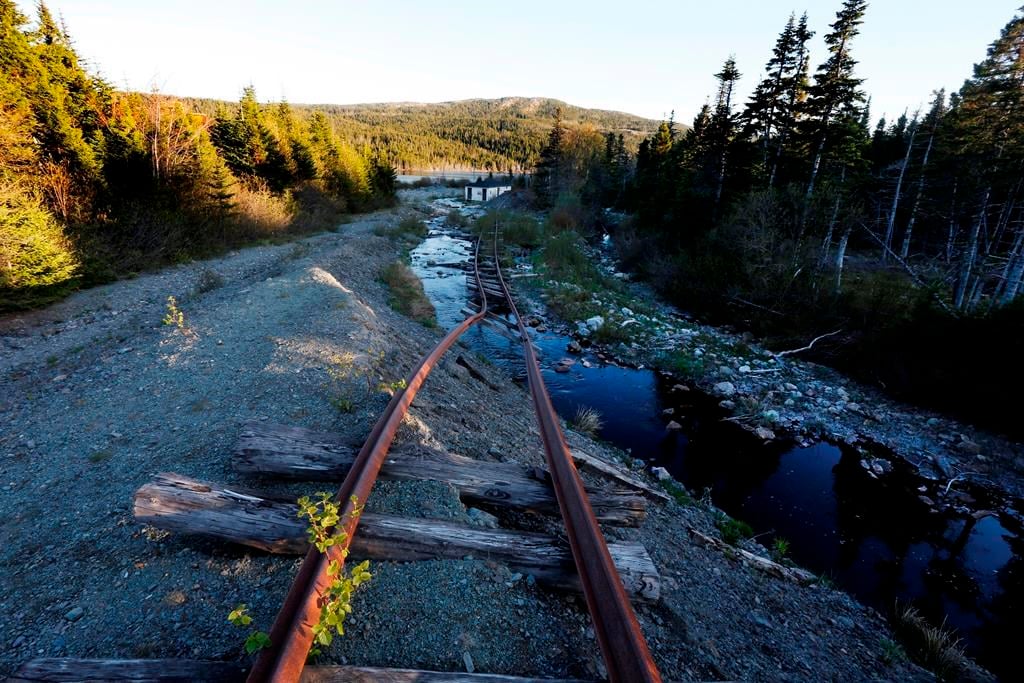The photograph captures an abandoned and neglected railroad track situated in a natural, outdoor setting during the daytime. The square, full-color image focuses on an old rail line descending from the bottom center and bending into a small, deep blue river, which is eroding the land and causing the remaining support logs to be washed away. The rails themselves are brown and rusted, clearly unusable. On the right-hand side, tall, green pine trees, some of which have dead, white branches, stand next to the river, accompanied by large white rocks and green bushes. On the left-hand side, shorter green pine trees are illuminated by sunlight. The upper portion of the image features a blue sky with rolling hills in the distance, dense with more pine trees. This photo emphasizes the remnants of an old railway amidst a vividly natural, somewhat wild landscape.